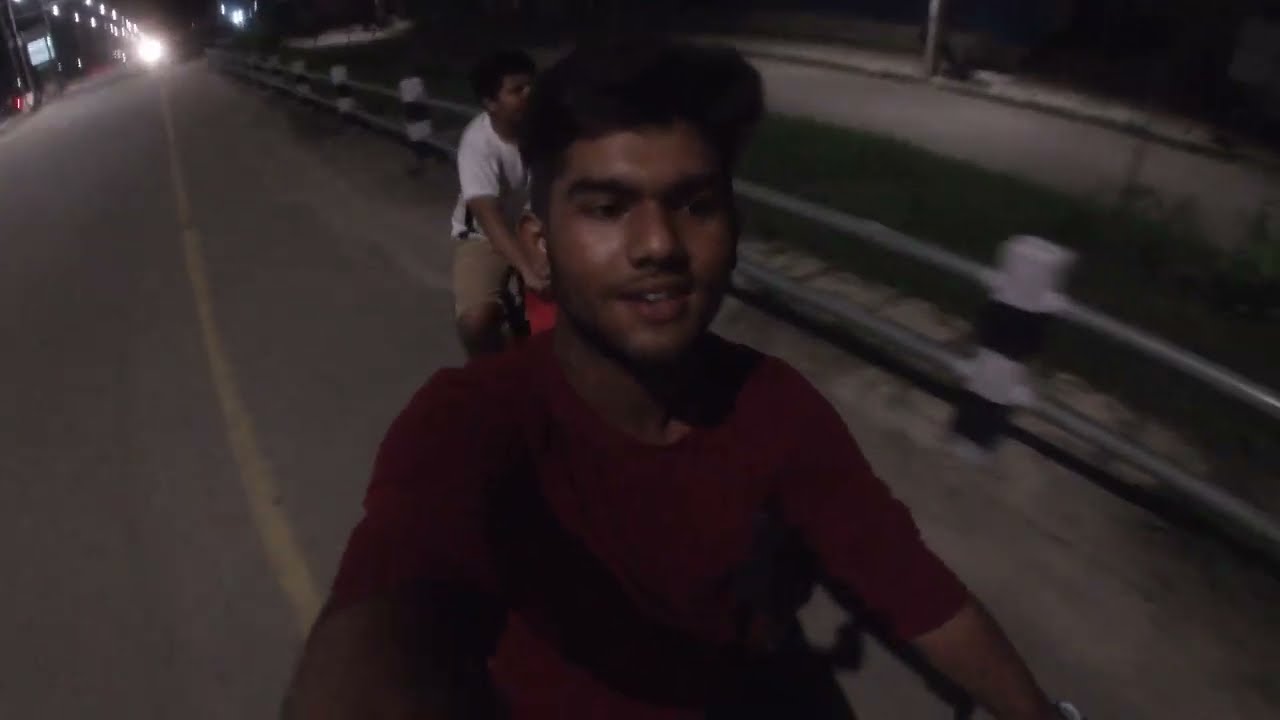The image captures a nighttime scene with two young, dark-skinned Indian men riding bikes along a road. The photograph is blurry, likely taken in motion, and shows the man closest to the viewer wearing a long-sleeve red shirt with the sleeves rolled up. He has black hair that poofs up in the front and is looking off to the right with a faint smile. He appears to be concentrating on riding his bike, which is not fully visible. Behind him, another man, also with dark hair, is riding a bike. This second rider is dressed in a white t-shirt and khaki pants. The setting is alongside a paved road with a yellow stripe, bordered by a silver guardrail with black and white pylons. Additional lights, presumably from passing cars, can be seen in the top left corner of the image.